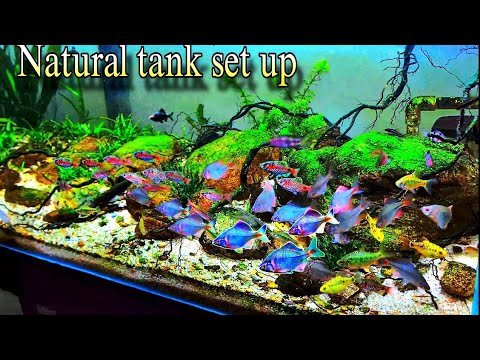The image showcases a vibrant aquarium labeled "Natural Tank Setup" in the top left corner, encased by a black border at the top and bottom. The tank, filled with vivid life, is dominated by bright green plants that stand out amidst fluorescent bright blue and smaller pink fish swimming on the right side. The bottom of the tank features light-colored gravel interspersed with various plants. In the background, a pipe and a stick or twig-like device are discernible in the top right corner, while what resembles a copper plumbing pipe is visible towards the back right. The aquarium is alive with movement and colors—from the gradient blue fish to the smaller yellow and reddish ones. The setting is enhanced by the presence of mossy rocks, branches, and barnacles, creating a visually captivating natural underwater environment.